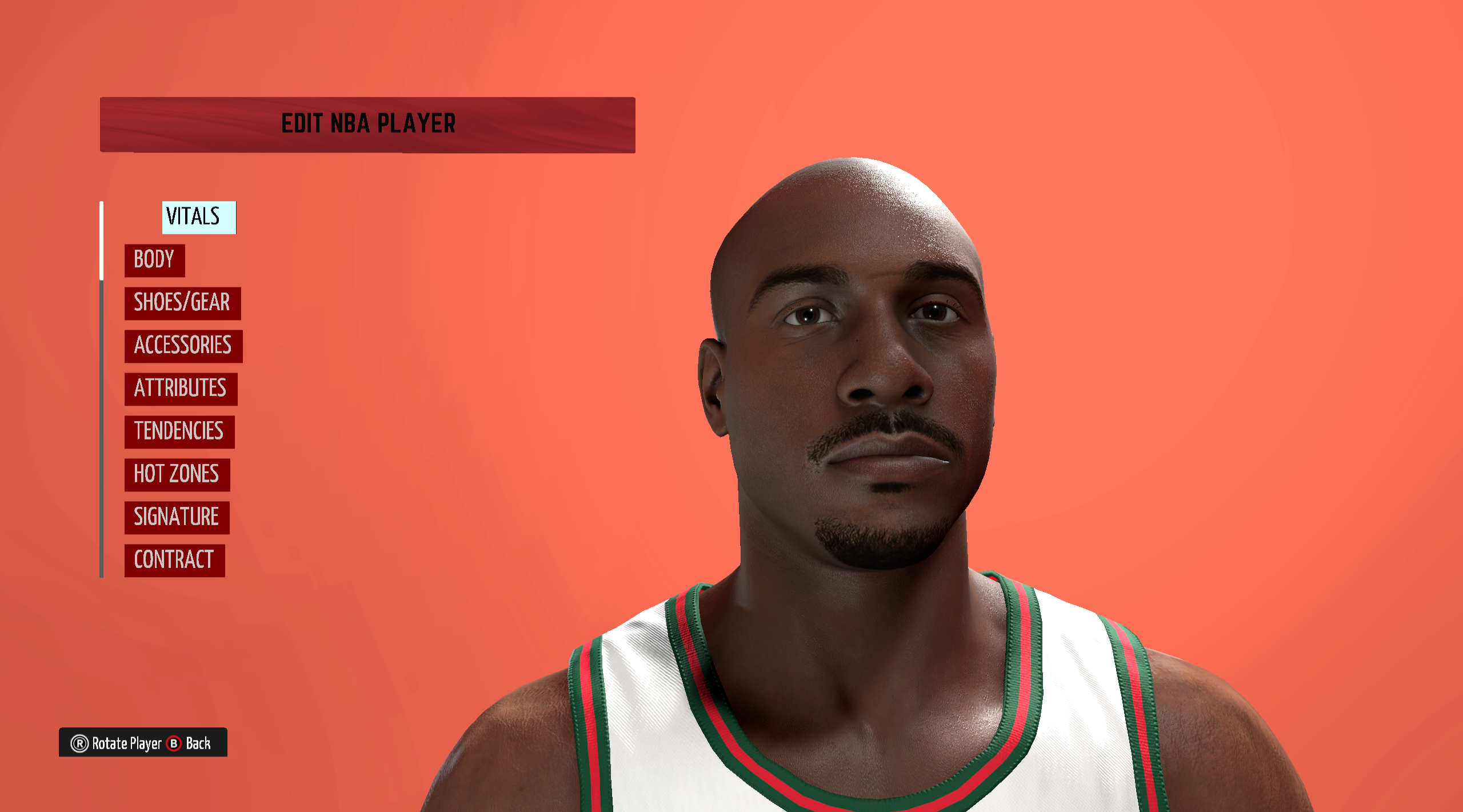The image features a lifelike AI-generated depiction of an African-American NBA player set against a vibrant, melon-colored backdrop that combines a striking blend of bright orange and magenta hues. The player is characterized by smooth dark skin, a bald head, thick eyebrows, dark eyes, and notable facial hair, including a mustache and goatee. Despite the realistic appearance, he's not smiling.

The player dons a pristine white sleeveless jersey accented with green and magenta trims along the collar and armholes, echoing the vivid tones of the background. Several interface elements, indicative of an AI editing program, are overlaid on the image. 

Noteworthy highlights in red blocks include: 
- "Edit NBA Player" in black text.
- "Vitals" positioned on the left side, within a white block with black text.

Additional customization options are listed, such as:
- Body
- Shoes
- Gear
- Accessories
- Attributes
- Tendencies
- Hot Zone
- Signature
- Contract

In the lower left corner, two black-labeled controls read "Rotate Player" and "Back." The overall composition is meticulous, bringing together detailed graphical elements that enhance the digital portrayal of the player.